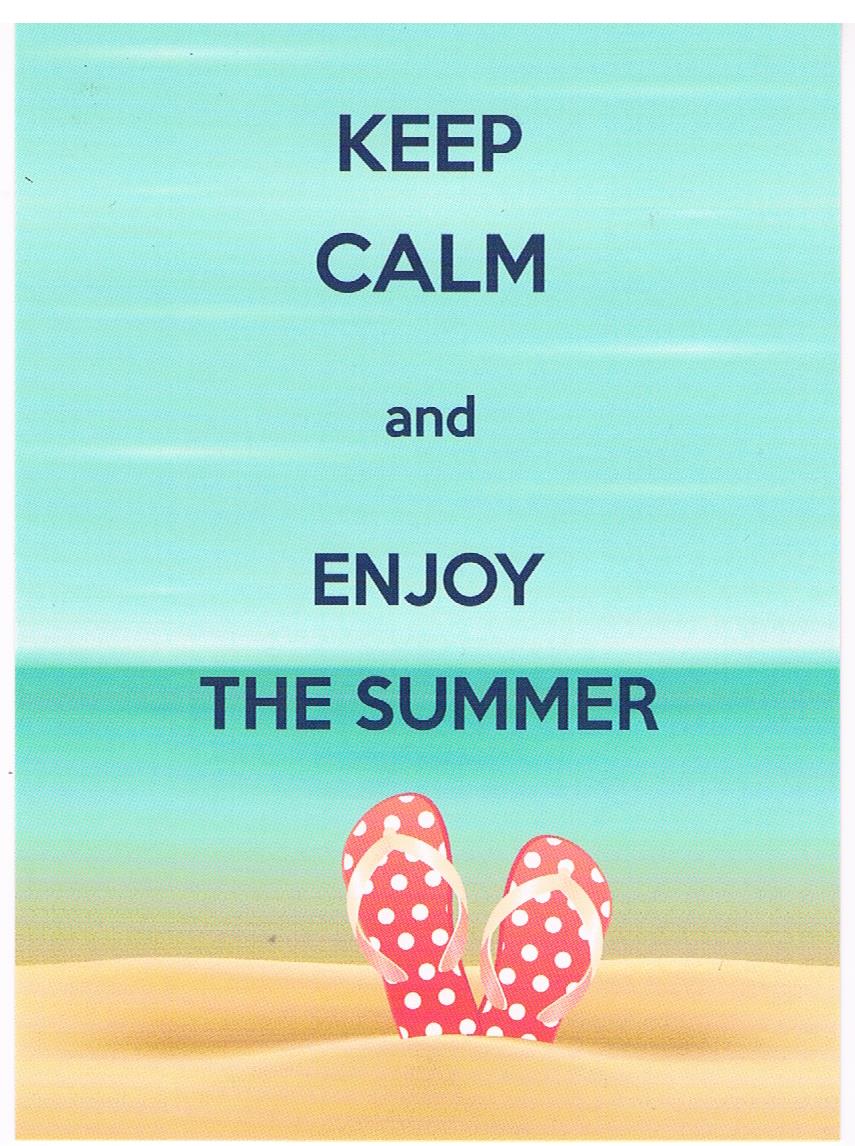The image is an illustration commonly seen on social media, portraying a tranquil beach scene with an inspirational message. The background is a gradient of greenish to light sky blue hues, resembling a watercolor effect, with soft, white streaks mimicking clouds. In the foreground, there is a yellow sandy beach. Sticking upright in the sand is a pair of red flip-flops, adorned with white polka dots and light pink straps. The middle section of the image represents a body of seafoam green water that blends into the sand and sky, creating a harmonious horizon line. At the top of the card, dark navy blue letters spell out the inspirational phrase: "KEEP CALM" in capital letters, followed by "and" in smaller, lowercase letters, and concluding with "ENJOY THE SUMMER" again in uppercase. The overall design evokes a peaceful, summery vibe, encouraging relaxation and enjoyment of the season.